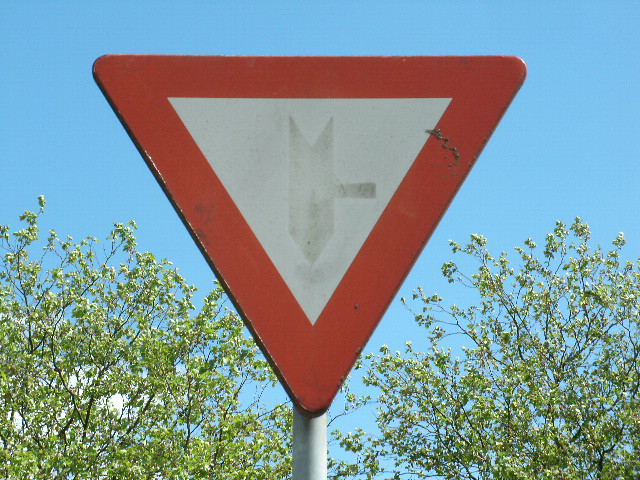The image depicts an old, weathered warning sign in the shape of an upside-down triangle. The sign features a red outline, with a white center housing a faded downward-pointing arrow. The background is a clear daytime setting, characterized by a bright blue sky and the sun shining overhead. Surrounding the sign are a few slender, vibrant trees with lush light green leaves. The ground in front of these trees is scattered with debris and dirt, adding to the aged appearance of the scene.